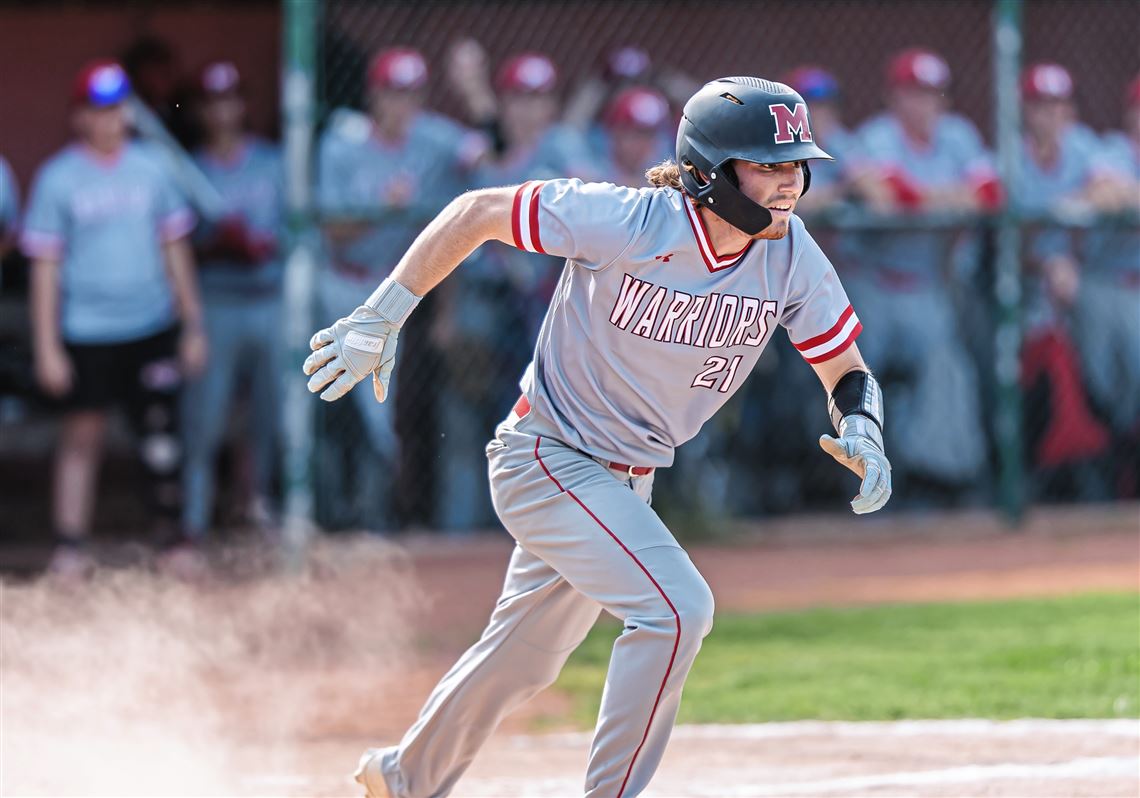The photograph captures an intense moment of a baseball game with a player, number 21 from the Warriors, running from first base to second base. Positioned at the center of the image, the athlete is clad in a light gray uniform detailed with red stripes—a red stripe runs down the pants while the armbands and neckband of the short-sleeved jersey are highlighted with red and white accents. His black batter's helmet prominently features a red M on the front, and the Under Armour logo is visible on his lapel. He is wearing gray batting gloves. The sun is shining brightly, casting shadows on the field, and the player is focused intently on the base ahead. In the background, the dugout is blurred but reveals around ten team members and a coach, all seemingly cheering him on. This high-quality, close-up image perfectly captures the quintessential energy and concentration of a baseball game.